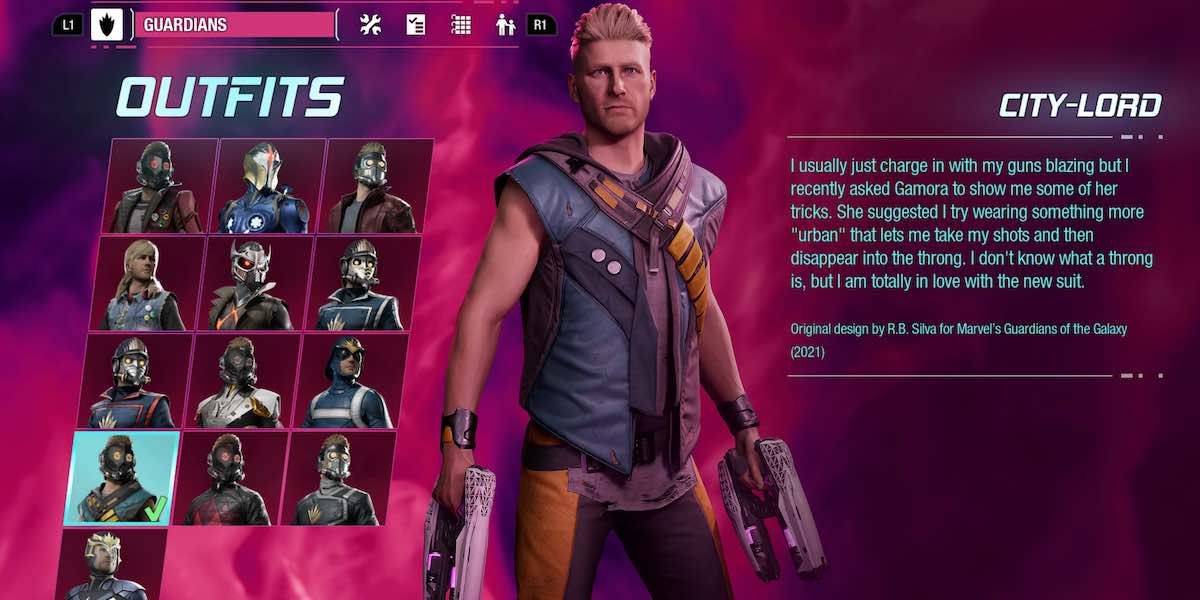The image depicts a loading screen from a video game, set against a smoky, hazy background of various shades of purple and pink. At the top of the screen, there's a search bar area labeled "Guardians" in pink, accompanied by several icons to its left: two wrenches, a checklist, a grid, and a figure representing an adult holding a child's hand. Below this, in large white letters, the word "Outfits" is displayed.

Under the "Outfits" title, a grid featuring 10 to 13 different characters or avatars is shown, each presumably wearing various outfits. Towards the right side of the screen stands a computer-generated male character with blond, slicked-back hair, dressed in a blue leather cut-off vest, leather pants, and wielding weapons in both hands. Adjacent to this character is a label in white font that reads "City Lord," identifying him as such. Below him, a teal text box contains the character's dialogue, explaining his change in attire based on advice from Dukamora. The message humorously notes his unfamiliarity with the term "throng" but expresses his satisfaction with his new urban suit. At the bottom of the screen, it mentions the original design credit: "R.B. Silva from Marvel's Guardian of the Galaxy," copyrighted in 2021.